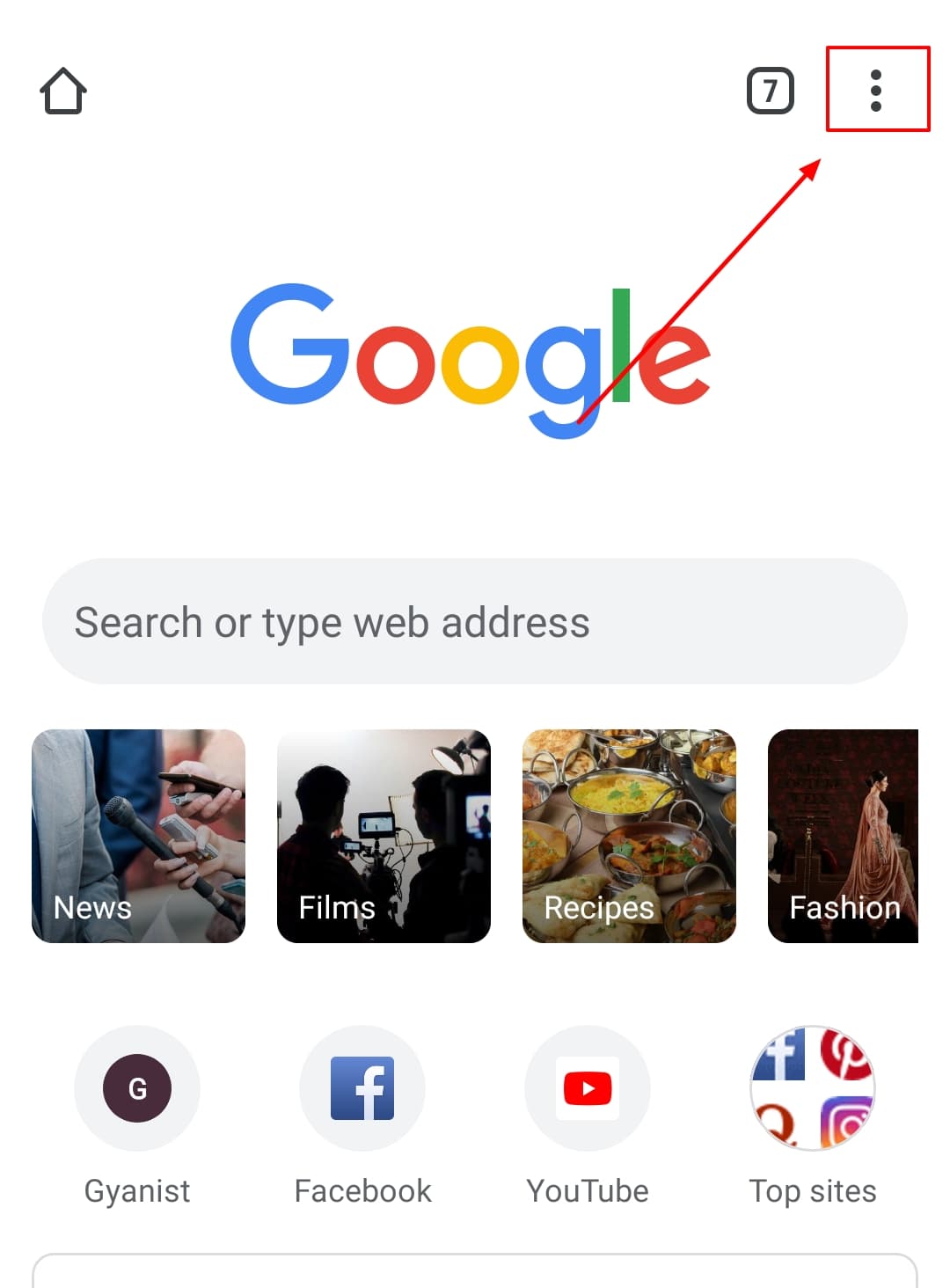This is an image of a Google search page with several notable elements highlighted. In the upper left corner is the Google home button, while on the right side, a red box and arrow draw attention to three vertically aligned dots, often indicating a settings or options menu. The search or type web address field is prominently displayed at the top. Below this are five tabs labeled "News," "Films," "Recipes," and "Fashion," each overlaid on a corresponding photograph; four photographs are fully visible, with one partially shown. Beneath these tabs, circular icons with the labels "Gynast," "Facebook," "YouTube," and "Top sites" are visible, though the view is cut off at the bottom. The background is predominantly white, with a variety of colors including blue, red, orange, yellow, and brown. The presence of the red box and arrow suggests an educational or instructional purpose, possibly explaining a feature related to the three-dot menu. Additional colors identified in the image include pink, a brownish-red, and silver.